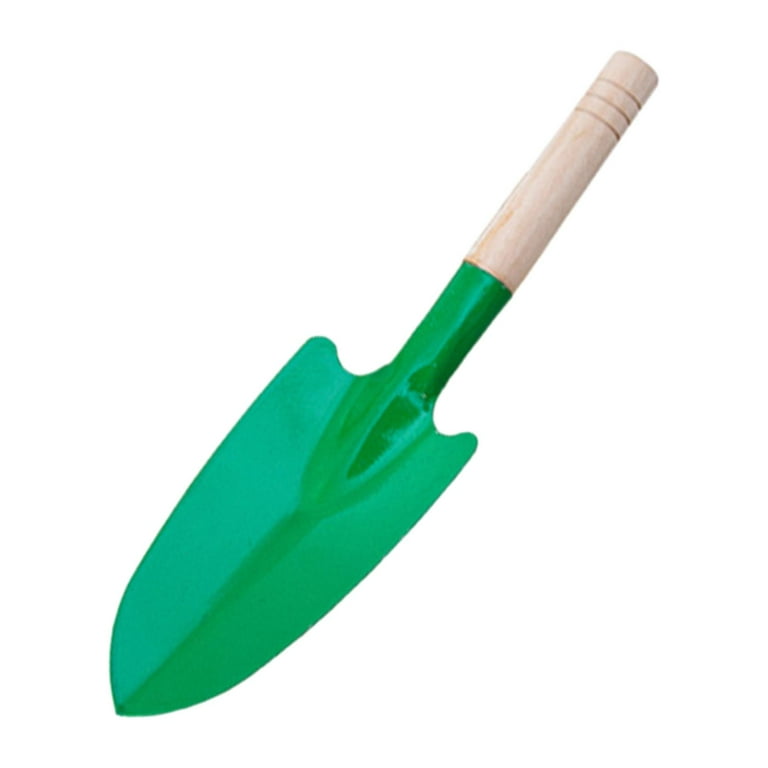The image depicts a gardening trowel displayed against a plain white background. The trowel features a short, pale wooden handle with three carved grooves near the top for a better grip. Attached to the handle is the trowel's blade, made of painted metal in a vibrant green color. The blade is concave, making it effective for scooping soil, and it tapers down into a pointed tip. The metal portion attaches to the handle with a straight section that curves inward in a circular hook-like fashion, reinforcing the connection between the blade and the handle.